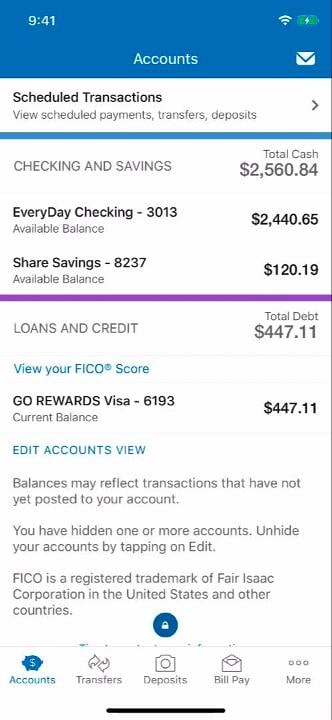This image depicts a smartphone screen displaying a banking application. 

In the top right corner, there are icons indicating wireless signal strength and battery status, with the battery currently charging. The top left corner shows the time as 9:41.

The screen's main header reads "Accounts," accompanied by an envelope icon on the far right. Below this, there is a section labeled "Scheduled Transactions," describing options for scheduling payments, transfers, and deposits.

Next is a section titled "Checking and Savings," showing a total cash amount of $2,560.84. It details two accounts: 
1. "Everyday Checking-3013" with an available balance of $2,440.65.
2. "Share Savings-8237" with an available balance of $120.19.

A purple horizontal line separates this section from the next, which is labeled "Loans and Credit." This section indicates a "Total Debt" of $447.11 and provides an option to view your FICO score. Specifically, it lists:
- "GoRewardsVisa-6193" with a current balance of $447.11.

At the bottom of this section, text notes that account balances may reflect transactions not yet posted and that one or more accounts are currently hidden. It advises users to tap "Edit" to unhide accounts. Additionally, it includes a disclaimer that FICO is a registered trademark of Fair Isaac Corporation in the United States and other countries.

There is also a circular icon with a padlock in the middle symbolizing security. 

Finally, at the very bottom of the screen, menu options are listed: "Accounts," "Transfers," "Deposits," "Bill Pay," and "More."